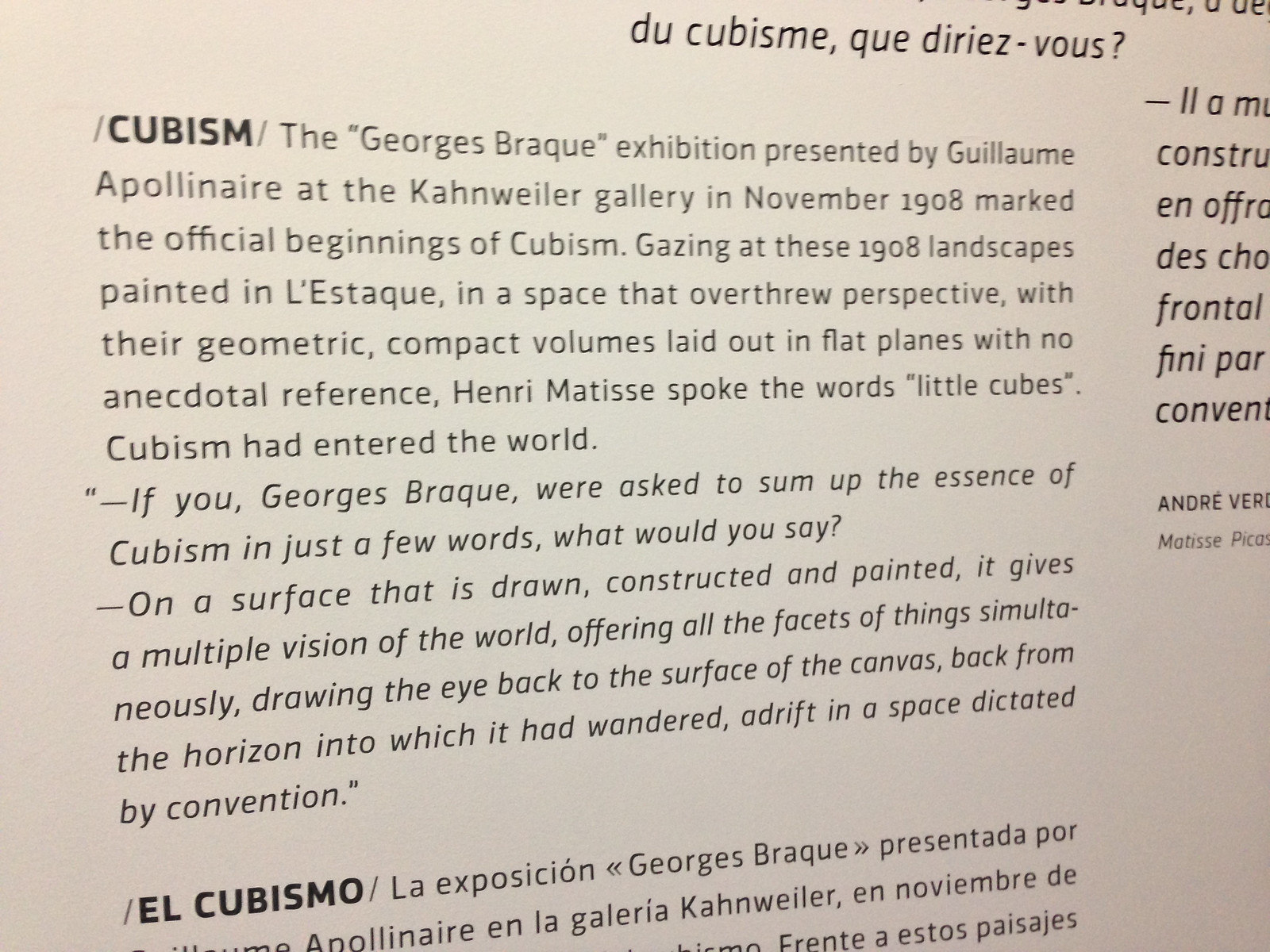The image depicts a close-up of a page, presumably from an art book or magazine, featuring a detailed discussion on cubism. At the top left, the page begins with the bolded word "CUBISM," followed by an explanation of its origins. The text in clear black font announces, "The Georges Braque exhibition presented by Guillem Apollinaire at the Conwayler Gallery in November 1908 marked the official beginnings of cubism." The passage continues to describe the impact of Braque's 1908 landscapes painted in L’Estaque, which introduced geometric compact volumes laid out in flat planes, devoid of anecdotal references. Notably, Henri Matisse's reaction to these paintings was quoted as, "little cubes," symbolizing the advent of cubism. Following this, there is a prominent quote by Georges Braque: "If you, Georges Braque, were asked to sum up the essence of cubism in just a few words, what would you say? On a surface that is drawn, constructed, and painted, it gives a multiple vision of the world, offering all the facets of things simultaneously, drawing the eye back to the surface of the canvas, back to the horizon into which it had wandered adrift, a space dictated by convention." The page also includes the text in Spanish and another partially visible quote on the right side.